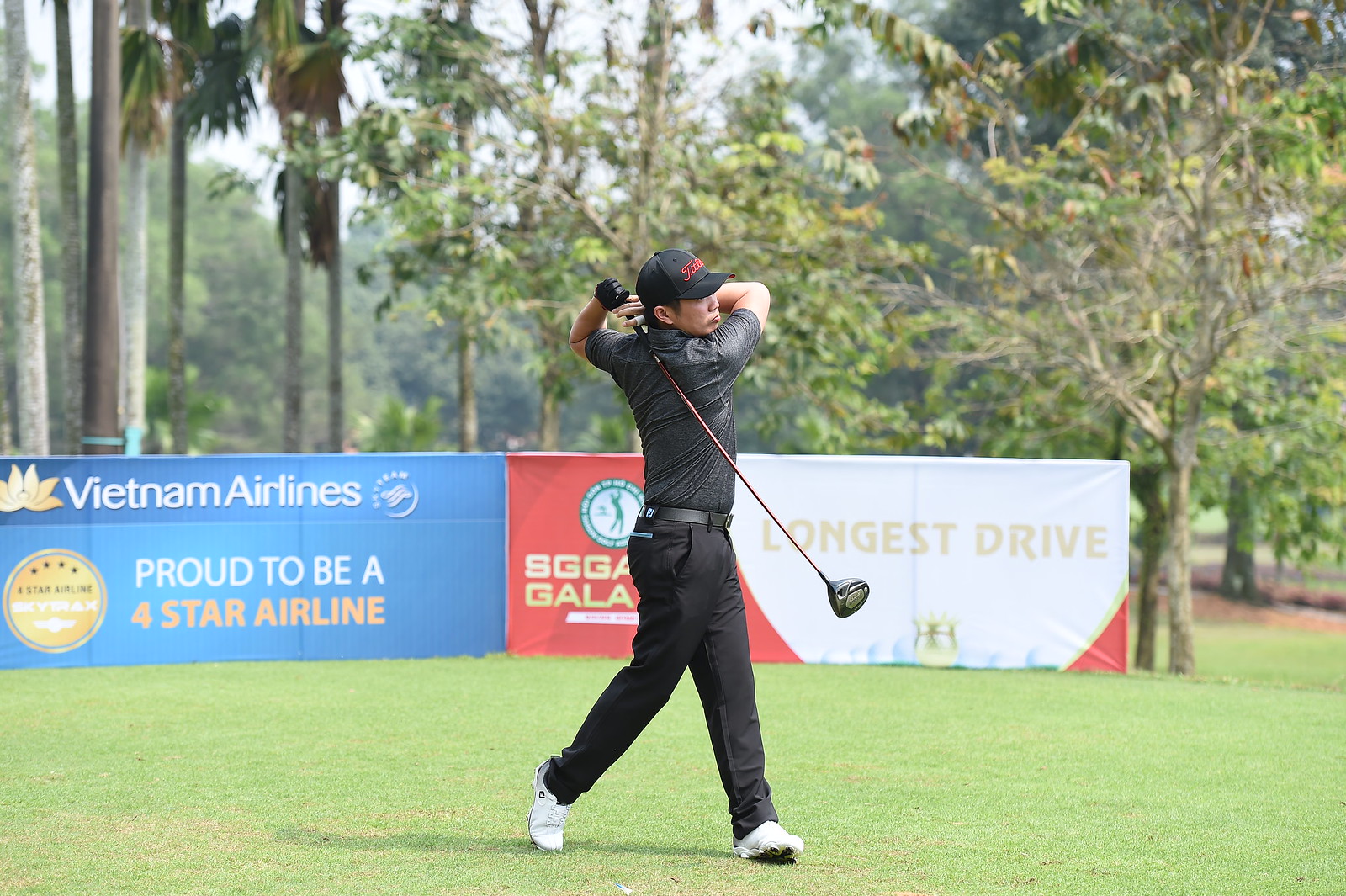In this detailed photograph, an Asian gentleman in his 30s or 40s is captured mid-golf swing on a lush green course, immediately after his drive. He is the sole subject of the image, dressed in black pants, a light gray short-sleeve polo shirt, white shoes, a black belt, and a distinctive black cap featuring a red Titleist logo. His hands are raised near his neck, indicating the completion of his powerful swing, and he wears a black glove on one hand. 

Behind him, a series of sponsorship banners add context to the scene, suggesting he is participating in a golf tournament. Prominent among these are a blue sign with white letters for Vietnam Airlines, boasting, "Proud to be a Four-Star Airline," and a red-and-white sign promoting the "SGG Gala Longest Drive." The backdrop also includes several trees, adding a natural, somewhat forested ambiance to the setting.